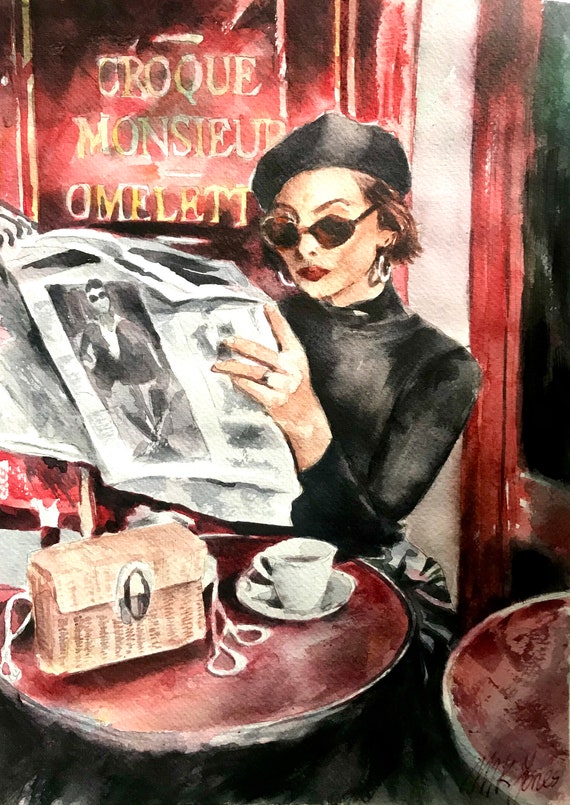This painting depicts a sophisticated woman seated in a French cafe, exuding an air of timeless elegance. Perched at a small red table, she has a tan and white rectangular purse placed beside a white mug of coffee on a matching white tray. The woman is stylishly dressed in a black turtleneck and a black beret, accessorized with brown sunglasses and vibrant red lipstick. Her poised left hand, adorned with a ring, holds up a black-and-white newspaper featuring a well-dressed man wearing black sunglasses on the cover. The ambiance is further enhanced by a red sign in the background displaying items such as "croque monsieur" and "omelette," confirming the quintessentially French setting of the cafe.